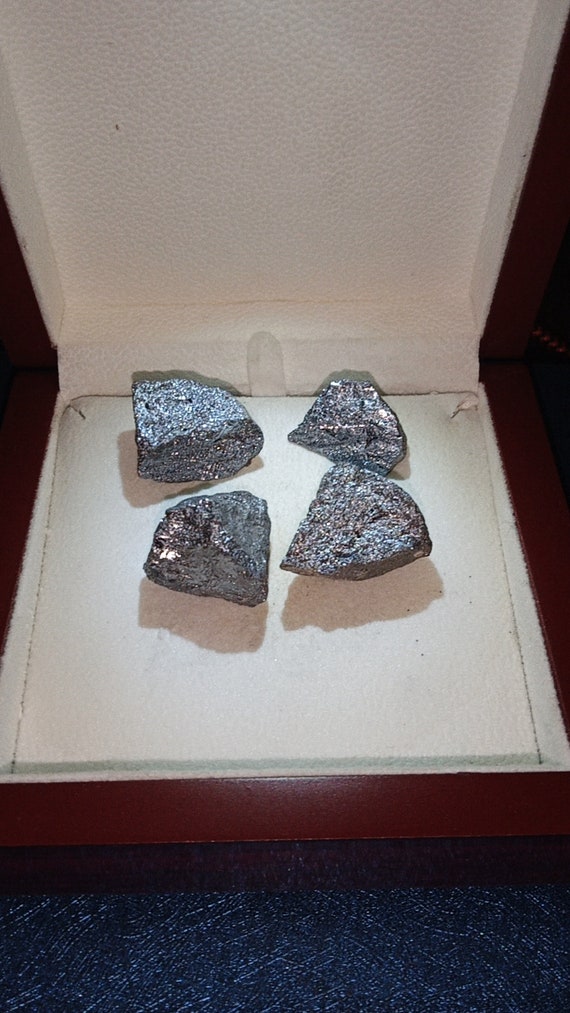This photograph features four small, silvery-gray rocks arranged neatly within an open display case. The display case, which has a wooden brown edge and a white interior likely resembling or covered in fabric, appears comparably similar to a large jewelry or ring box. The four stones, which are described as shiny and plain, with no particularly notable features, are positioned with two on the top and two on the bottom. The entire setup rests on a dark blue or black table or mat, providing a contrast to the lighter colors of the display case and the stones.